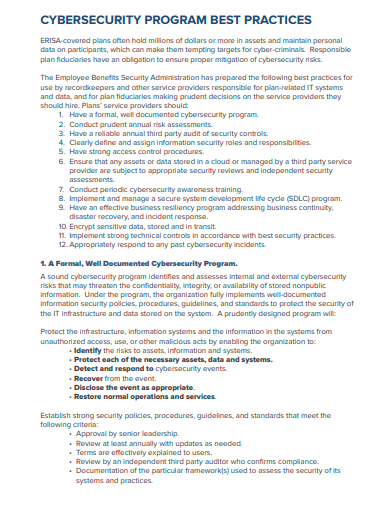**Screenshot of Cybersecurity Program Best Practices on a White Background**

The screenshot captures the top section of a webpage with its background in white, featuring vibrant, multi-colored text. At the very top, from left to right, there is a prominent header in bold black letters: "Cybersecurity Program Best Practices." Just below this header, smaller gray text reads: 

"ERISA-covered plans often hold millions of dollars or more in assets and maintain personal data on participants, which can make them tempting targets for cyber criminals. Responsible plan fiduciaries have an obligation to ensure proper mitigation of cybersecurity risks."

Further down, additional gray text states:

"The Employee Benefits Security Administration has prepared the following best practices for use by record keepers and other service providers responsible for plan-related IT systems and data, and for plan fiduciaries making prudent decisions on the service providers they should hire."

Below this introduction, there is a numbered list (1 through 12) detailing specific best practices:

1. Have a formal, well-documented cybersecurity program.
2. Conduct prudent annual risk assessments.
3. Have a reliable annual third-party audit of security controls.
4. Clearly define and assign information security roles and responsibilities.
5. Have strong access control procedures.
6. Ensure that any asset or data stored in a cloud or managed by a third-party service provider is subject to appropriate security reviews and independent security assessments.
7. Conduct periodic cybersecurity awareness training.
8. Implement and manage a security system development life cycle (SDLC) program.
9. Have an effective business resiliency program addressing business continuity, disaster recovery, and incident responses.
10. Encrypt sensitive data both stored and in transit.
11. Implement strong technical controls in accordance with best security practices.
12. Appropriately respond to any past cybersecurity incidents.

Following this list, there is an additional paragraph labeled as item number one, with a bold black heading: “A formal, well-documented cybersecurity program.” The accompanying detailed description outlines:

"A sound cybersecurity program identifies and assesses internal and external cybersecurity risks that may threaten the confidentiality, integrity, or availability of stored nonpublic information. Under the program, the organization fully implements well-documented information security policies, procedures, guidelines, and standards to protect the IT infrastructure and data stored on the system. A prudently designed system will:"

This description is followed by a series of six bulleted items, each starting with a bold black keyword:

- **Identify**: the risks to assets, information, and systems (in gray text).
- **Protect**: each of the necessary assets, data, and systems.
- **Detect and respond**: to cybersecurity events.
- **Discover**: from the event.
- **Disclose**: the event as appropriate.
- **Restore**: normal operation and services.

These detailed best practices serve as guidelines for enhancing the cybersecurity measures of organizations managing ERISA-covered plans and other sensitive information.